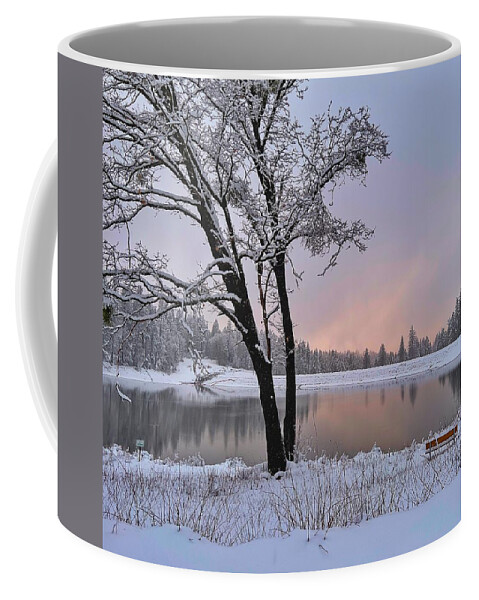In the photo, there is a giant coffee mug set against a white background, featuring a white handle and a grayish interior. The mug showcases a detailed and scenic winter landscape. The image on the mug depicts a frozen pond surrounded by snow-covered ground and trees stripped of their leaves. Despite the cold, a vivid rainbow arcs through the hazy skies, which could be mistaken for northern lights at sunrise or sunset, emanating colorful rays above the pine trees at the horizon. The foreground features a solitary bench and an oak tree at the edge of the snow-encircled pond. The serene winter scene is devoid of people or animals, though there is a possible avian silhouette in the bottom left corner, which might be a swan or crane, blending into the snowy environment.